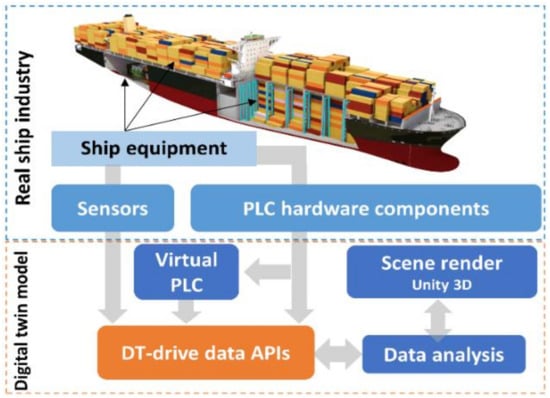This is a detailed diagram of a large cargo ship, divided into two main sections, each outlined in a distinct color. The top half, enclosed by a blue-dotted rectangle, is labeled "Real Ship Industry" in black text. Central to this section is a cutaway illustration of a cargo ship, revealing multicolored cargo containers—yellow, red, blue, white, and orange—stacked between aqua blue beams. The ship features a white tower at its center with a green object on top, tilting outward on either side. The visible hull of the ship is black on top with a continuous black stripe, while a red stripe runs along the bottom.

Three black arrows originating from the label "Ship Equipment" on a blue background point to different sections of the ship—the rear, middle, and top. Attached to "Ship Equipment" are gray arrows that branch out to two dark blue boxes labeled "Sensors" on the left and "PLC Hardware Components" on the right.

Below this, occupying the bottom section and defined by an orange-dotted outline, is the "Digital Twin Model." Here, arrows from the top section lead into a blue box labeled "Virtual PLC," which then directs to an orange rectangle titled "DT Drive Data APIs." Two-way gray arrows extend from this rectangle to two blue boxes: one labeled "Data Analysis" and the other "Scene Render Unity 3D." Along the far left edge of the bottom half, the term "Digital Twin Model" is written vertically in black letters. The entire diagram effectively illustrates the interconnected components and data flow of a cargo ship within the ship industry and its digital twin model.